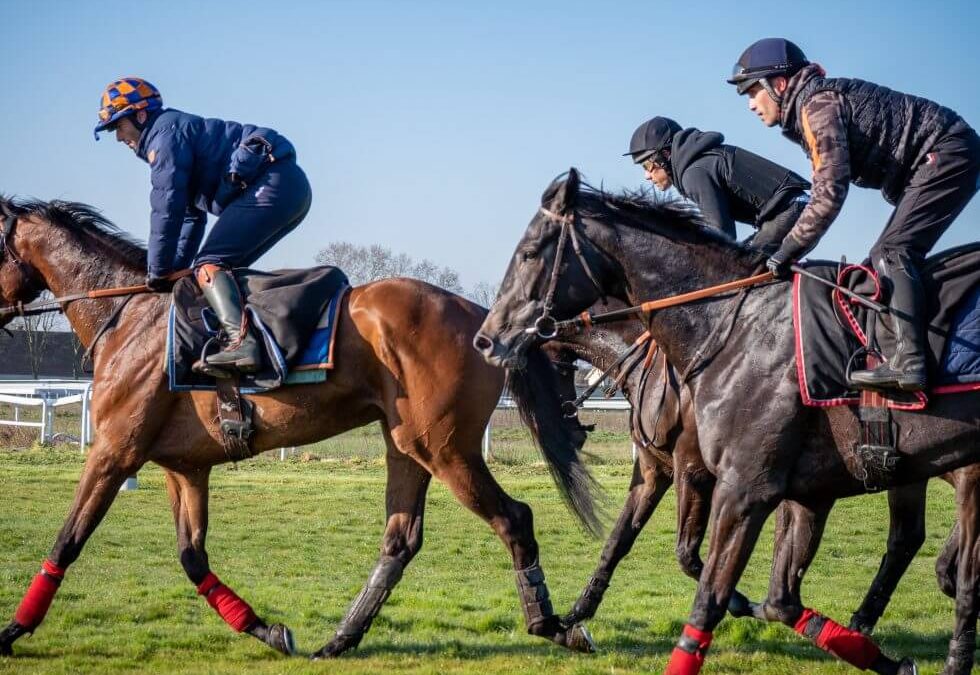The image portrays three men, visibly jockeys, riding horses across a vibrant green grassy field under a blue sky. The men are semi-crouched in their stirrups, indicating that they are in motion. 

The lead jockey is on a light bay horse, donning blue jodhpurs, black riding boots, and a blue puffer jacket. His helmet is uniquely patterned with orange and blue checks. His horse is adorned with red wraps around its front legs and black ones on its hind legs. 

Behind him, two other jockeys ride darker bay horses. The second jockey, visible in an orange and gray long-sleeved shirt under a black vest and a blue helmet, rides a horse with only its legs visible. The third jockey wears a navy blue sweatshirt and black helmet; his horse’s head is not in the frame.

All three men, presumed to be white, navigate the field with minimalistic saddles—essentially blankets with stirrups, and each firmly grips the reins. A traditional white picket fence outlines the lush field, adding to the picturesque setting.